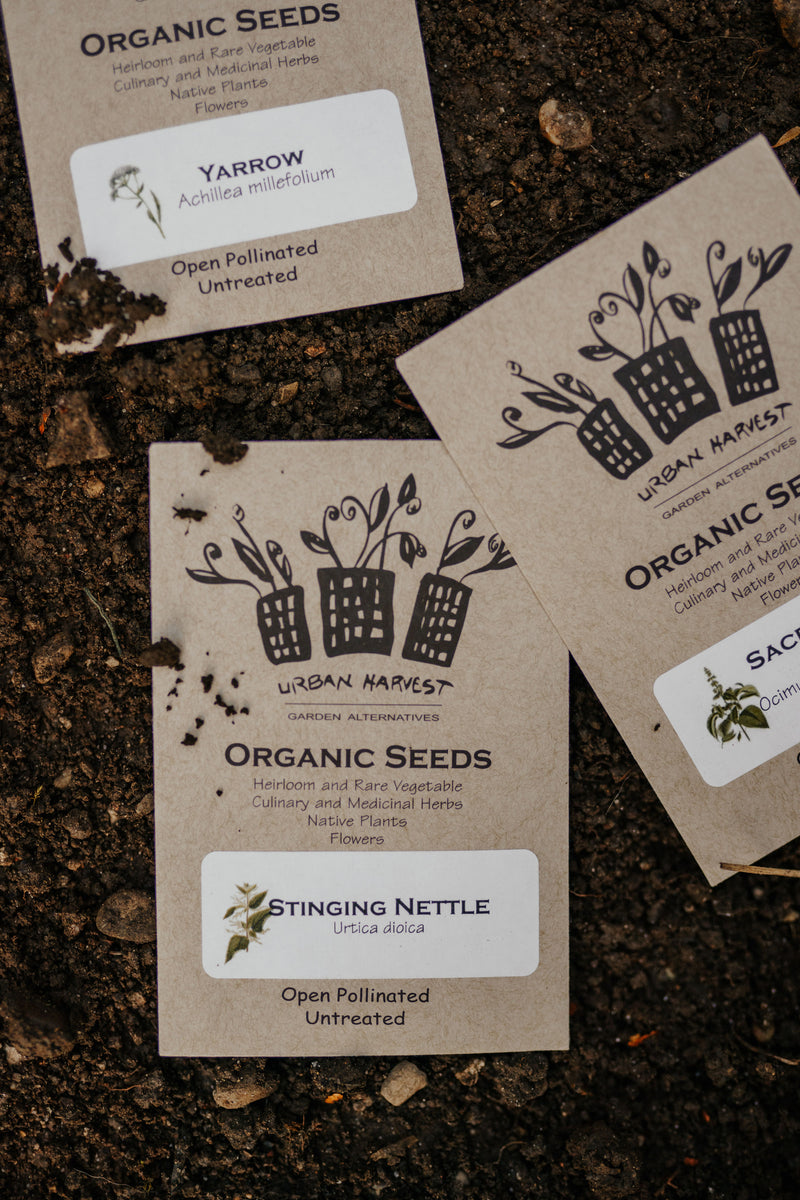This outdoor photograph features three brown packets of organic seeds from Urban Harvest, lying on a dark soil surface mixed with stones. Each packet displays black graphics of three pots with plants growing out of them. The text reads, "Urban Harvest Garden Alternatives Organic Seeds, Heirloom and Rare Vegetable, Culinary and Medicinal Herbs, Native Plants and Flowers." The central packet is labeled "Stinging Nettle (Urtica dioica), Open Pollinated Untreated." The packet to the left is for "Yarrow (Achillea millefolium)," while the packet to the right, slightly angled and partially cut off, starts with "SAC" and "OCIM," indicating another plant variety. Some soil has spilled over the packets, enhancing the earthy setting.